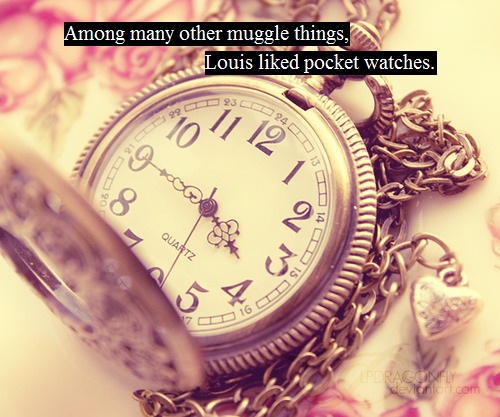The image appears to be a close-up shot of a beautifully ornate, gold pocket watch adorned with a heart-shaped keychain on its chain. The pocket watch, which looks like it's straight out of a vintage collection, is open to reveal its detailed clock face, meticulously marked with numbers from 1 to 12. The current time displayed on the watch is 3:45. The photograph is filtered with a pink and yellow hue, adding a warm and nostalgic feel to the scene. Above the watch, metallic text reads: "Among many other muggle things, Louis liked pocket watches," suggesting a possible connection to the Harry Potter universe, given the mention of "muggles."